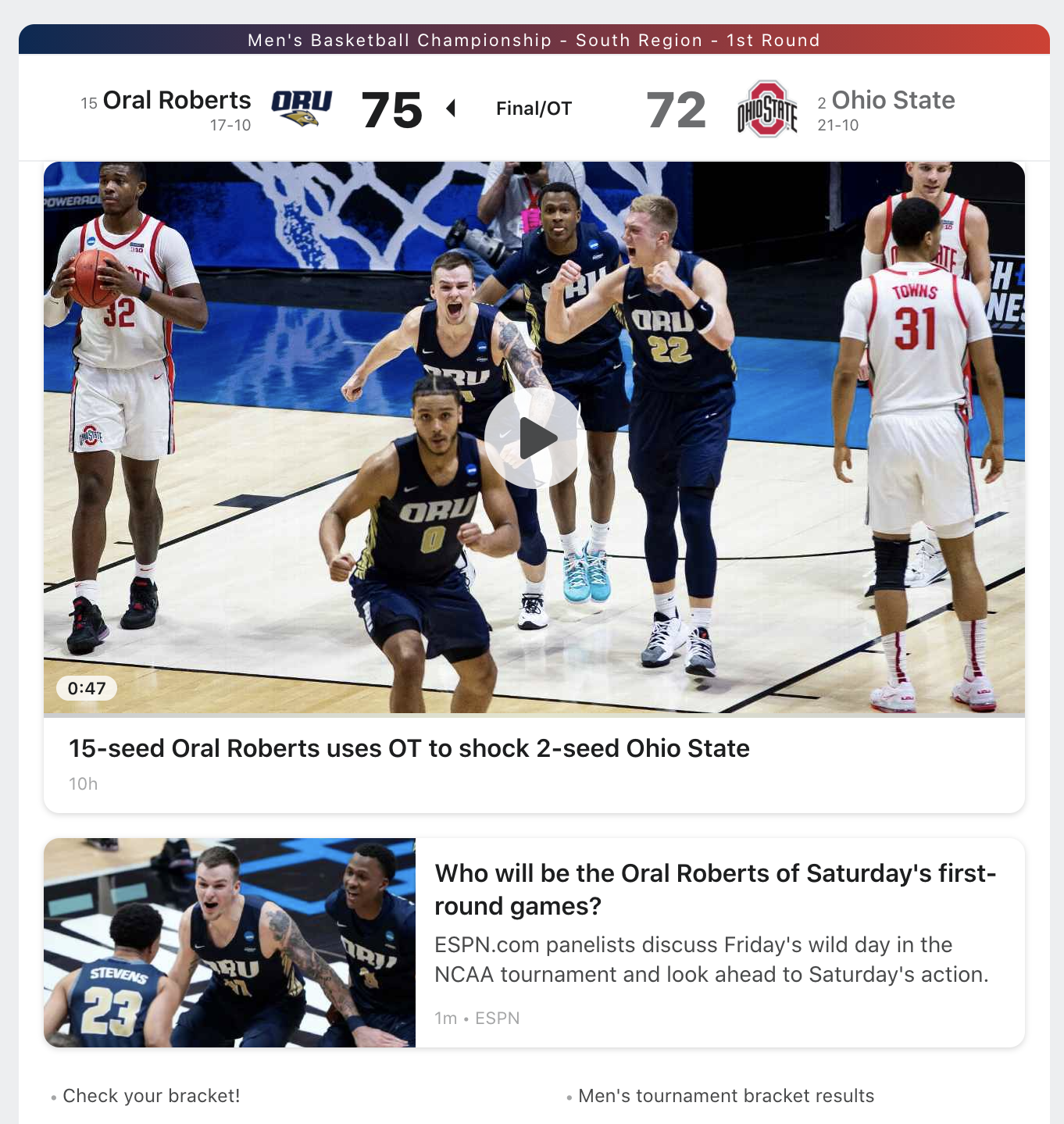This is a color image resembling a web page layout with a light grey border. Dominating the top of the image is a gradient banner that transitions from blue to red, featuring white text that reads: "Men's Basketball Championship, South Region, First Round." Directly below it lists the final overtime score: "Oral Roberts (ORU) 75, Ohio State 72."

A prominent photo or video thumbnail occupies the central portion of the image. This thumbnail depicts a basketball game in action, with a play button icon overlaid, suggesting that it is a video. The left and right edges of the thumbnail show players wearing white uniforms with red numbers, while the center features players in blue uniforms with "Opal" written on them and yellow numbers.

Beneath the video thumbnail, bold text states: "15 seed Oral Roberts uses OT to shock 2 seed Ohio State." There is another smaller image of basketball players to the lower left, next to a block of text on the right. This text reads: "Who will be the Oral Roberts of Saturday's first round games? ESPN.com panelists discuss Friday's wild day in the NCAA tournament and look ahead to Saturday's action."

At the bottom of the image, the left side offers an option to "Check your bracket," while the right side displays "Men's Tournament bracket results." A repeated line of text below the primary photo reiterates the headline, emphasizing the unexpected victory: "15 seed Oral Roberts uses OT to shock 2 seed Ohio State."

The image serves as a detailed snapshot of the game and provides context about Oral Roberts' surprising win over Ohio State in the NCAA tournament.